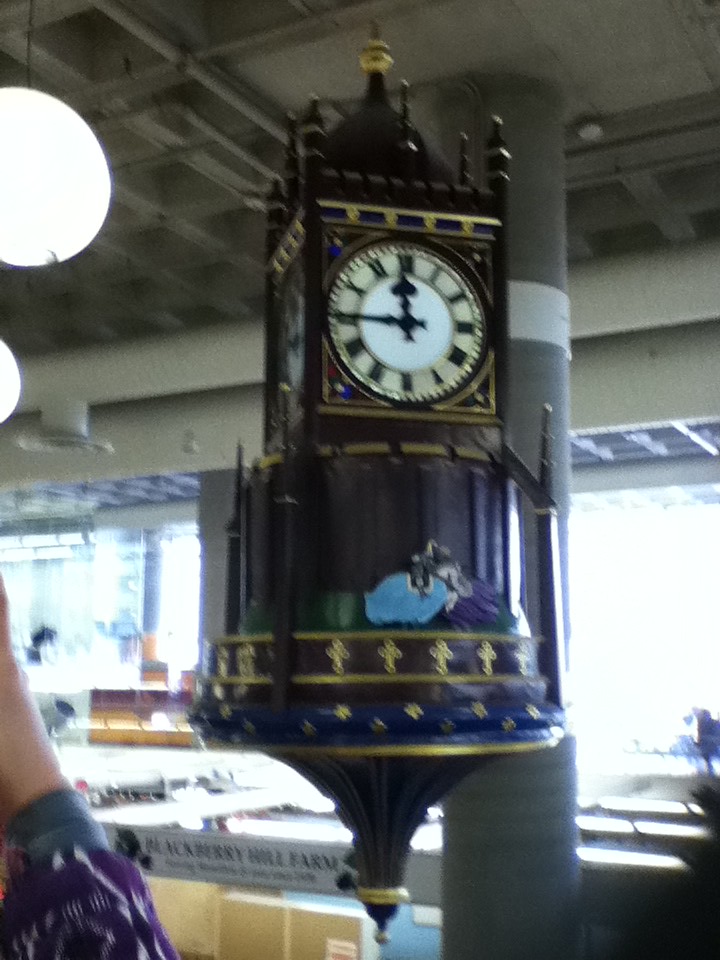The image depicts a slightly blurry, color snapshot taken inside a brightly lit building with visible ducting and ceiling tiles. In the center stands an elaborate, ornate clock. The clock has a square top, resembling a miniature version of Big Ben with spires and a pointed roof, adorned with Roman numerals on its faces. The clock appears to be brown with gold edges. Below the square portion is an upside-down, bucket-like shape leading to a spiraled decoration pointing downward. To the right, a woman's arm dressed in a purple and white sleeve is visible, indicating a person present in the scene. Behind the clock, bright sunlight streams through large windows, illuminating the area. The background includes metallic air conditioning pipes and the phrase "Blackberry Hill Farm" on a white rectangular sign, though it is somewhat blurry and hard to read.